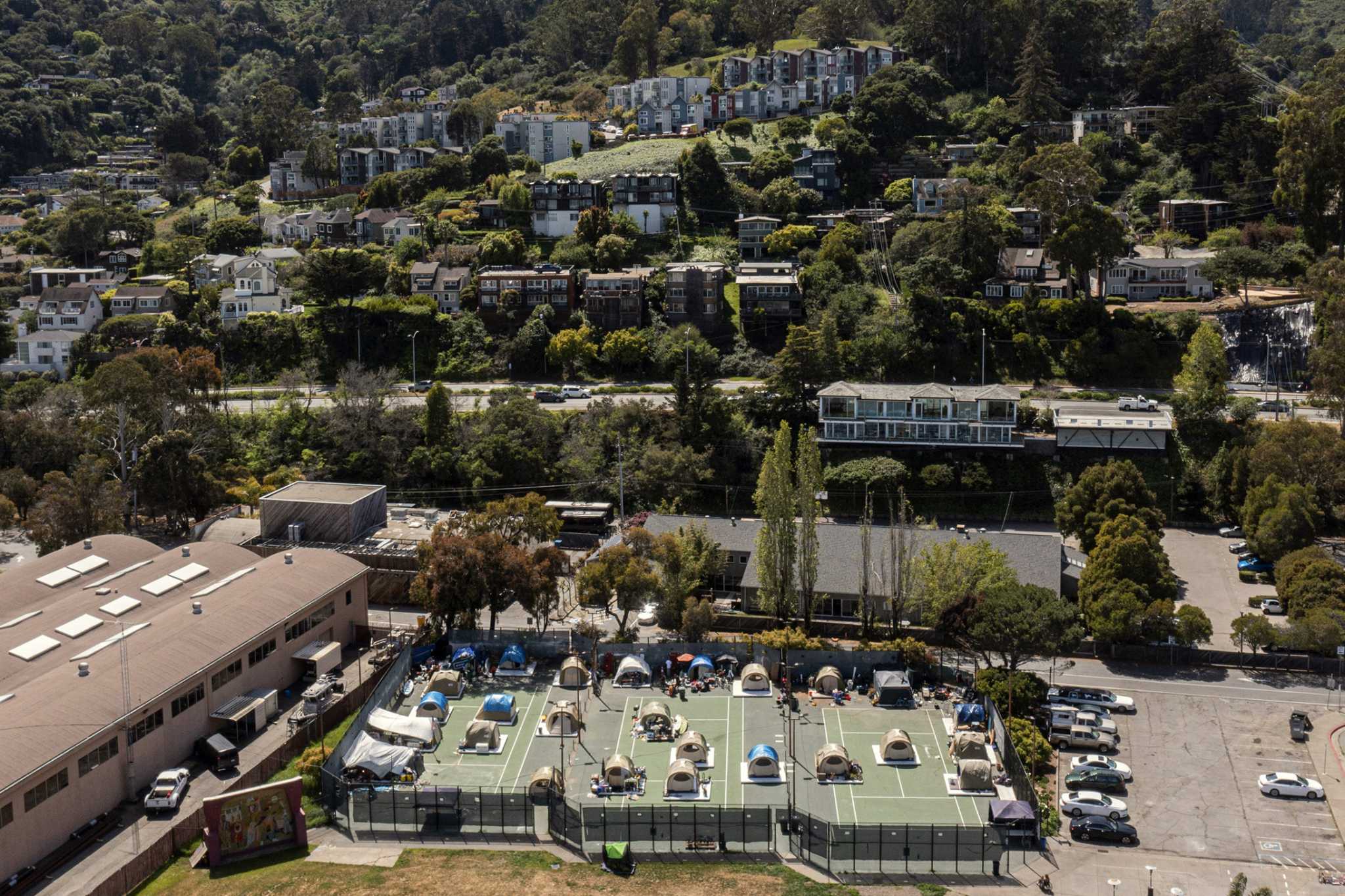The image is a color photograph captured from a bird's-eye view, possibly by a drone, showcasing a vivid and detailed layout of a small town or neighborhood on a sunny day. The scene prominently features a field in the front with numerous small tents set up, perhaps indicating a temporary encampment or shelter, which could be for homeless individuals or immigrants. To the right of the field is a parking lot, and to the left, a building of some sort is visible. The background of the image is filled with a variety of houses and small buildings, including some with balconies, spread out across a lush, tree-lined landscape. The overall setting appears vibrant and bustling with life, possibly suggesting a location like California.